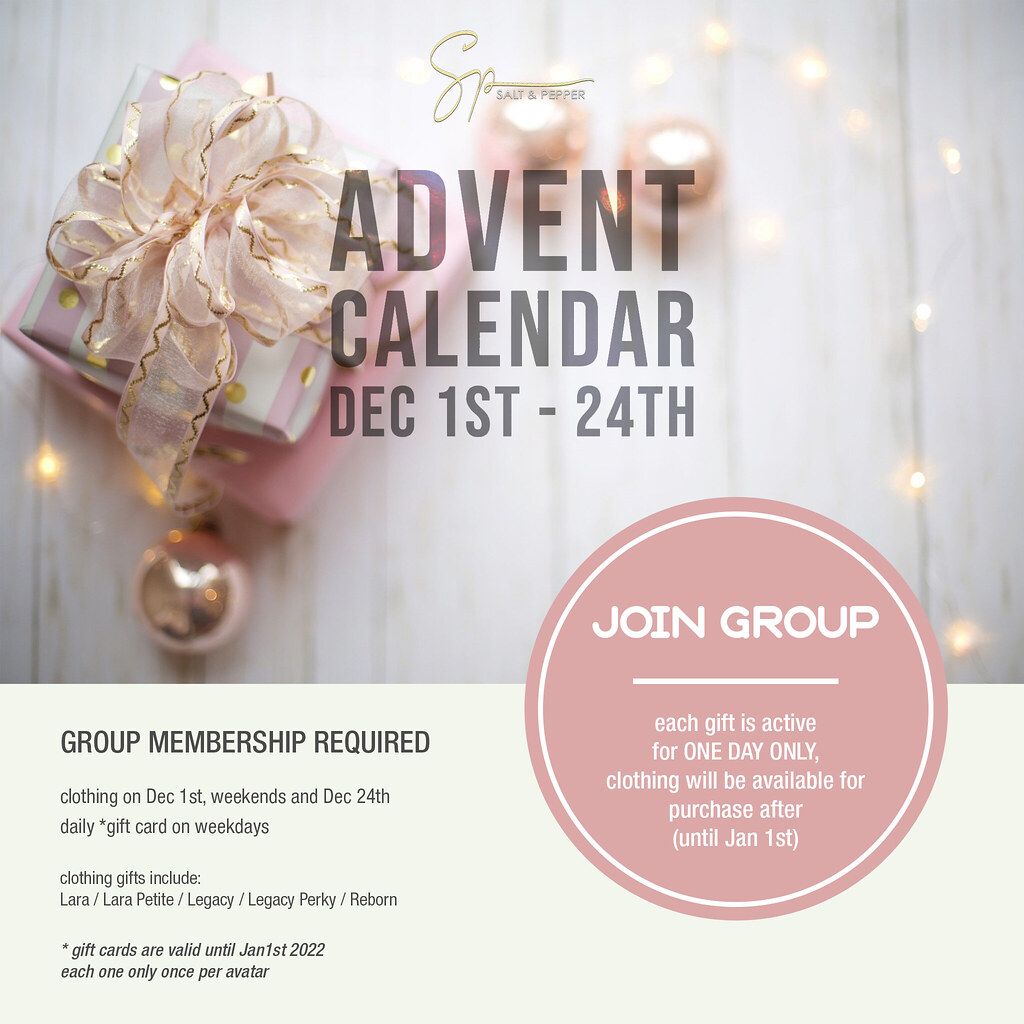This is a Christmas advertisement for an event by Salt and Pepper (SP) featuring an Advent Calendar running from December 1st to the 24th. The upper portion of the ad displays a slightly blurred, top-down view of a white wooden table adorned with two pink-wrapped gift boxes topped with bows, surrounded by three Christmas ornaments and festive fairy lights. The photograph is reminiscent of a vintage setup. The ad's text includes the title "Advent Calendar December 1st to 24th," prominently displayed at the top, followed by a pink circle in the bottom-right quarter with "Join Group" in white letters. Details on the promotion highlight that group membership is required. Clothing items are available on December 1st, weekends, and December 24th, with daily gift cards on weekdays. Each gift is active for one day only and clothing will be available for purchase until January 1st, 2022. The included clothing gifts are titled Laura, Laura Petit, Legacy, Legacy Perky, and Reborn. Gift cards can be used until January 1st, 2022, and each one can be redeemed only once per avatar.